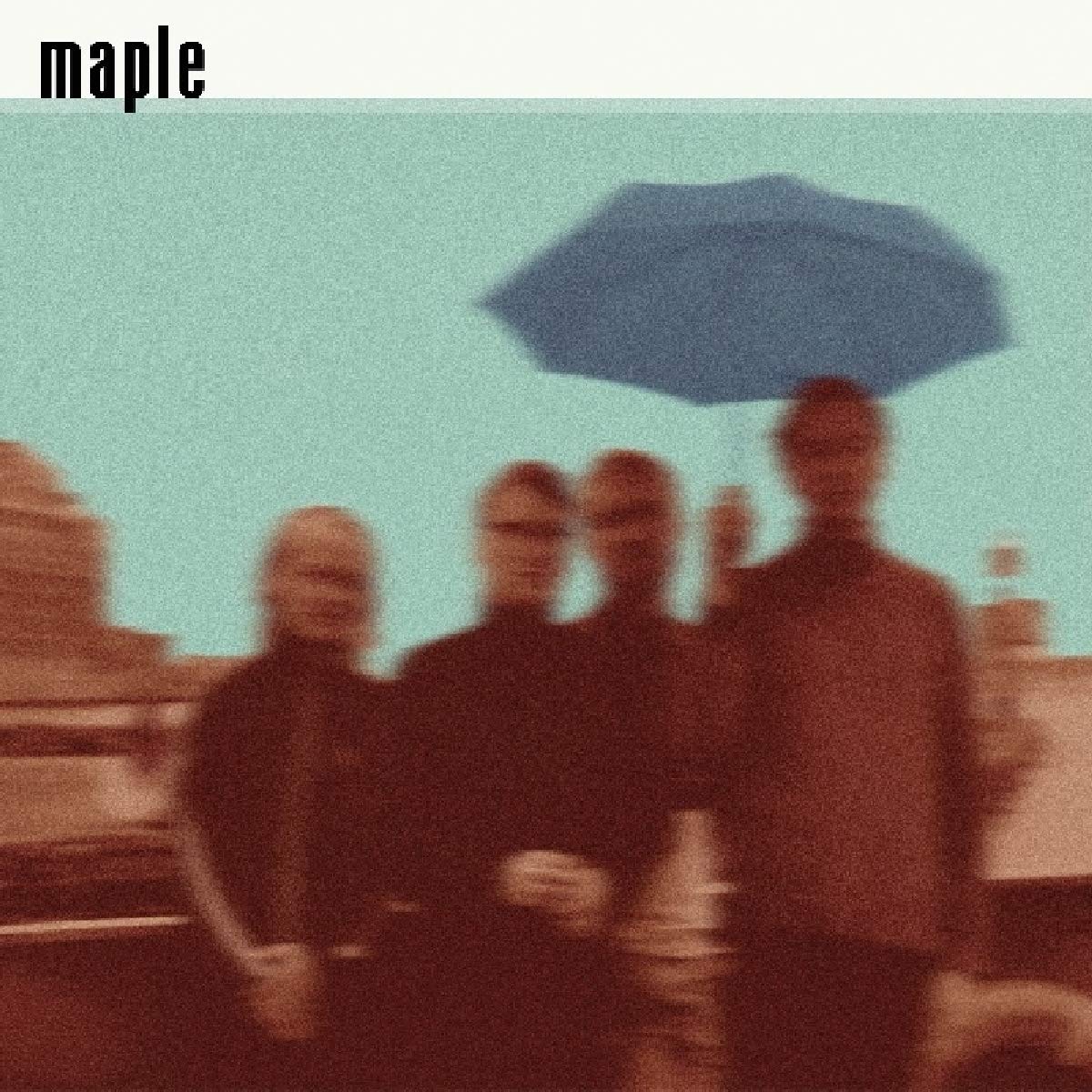This very blurry image appears to be an album cover with a turquoise-tinted sky in the background. In the upper left corner, outside the photograph, the word "Maple" is printed in black, presumably both the band name and the album title. In the center of the image, four young Caucasian individuals are standing. The woman on the far left has brown hair and is slightly shorter than the three men beside her. The two men in the middle are of similar height and both wear glasses. The man on the far right, who is the tallest, holds a blue umbrella above his head. All four appear to be just looking at the camera without much expression. The background on the left side features a building or possibly a brownish-red canyon-like formation, with a wall that has a handle running along it. The image overall has a rural feel, and its reddish tint adds to the vintage or stylized appearance.